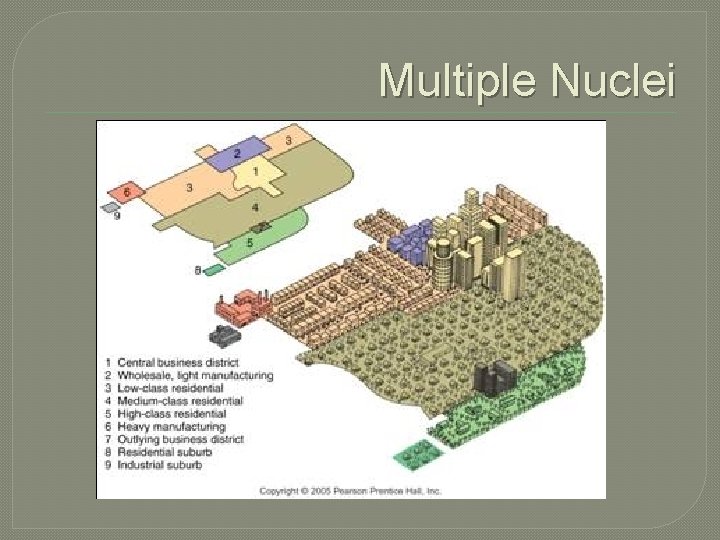This image is a detailed color-coded infographic styled like a PowerPoint presentation, centered perfectly in the photo. The central feature is a diagram resembling a Lego structure, illustrating various residential and manufacturing regions. The diagram is color-coded and numbered from 1 to 9, with each number representing different zones: Central Business District, Wholesale, Light Manufacturing, Low Class Residential, Medium Class Residential, High Class Residential, Heavy Manufacturing, Outlying Business District, Residential Suburb, and Industrial Suburb. These areas are marked in distinct colors including gray, brown, orange, pink, purple, green, tan, black, and white, and are identified by a detailed legend on the bottom left. At the top right of the infographic, "Multiple Nuclei" is prominently displayed in white font with a black drop shadow on a dark gray background. The bottom of the image includes black text indicating copyright 2005 Pearson Prentice Hall, Inc.